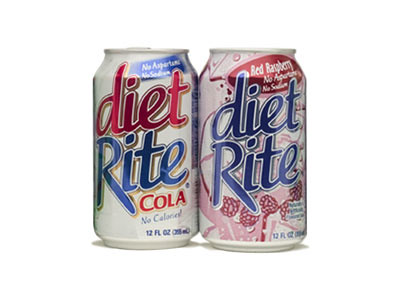The photograph features two cans of Diet Rite Cola placed side-by-side against a pristine white background, with a subtle shadow cast at the base of each can. The left can prominently displays "Diet" in bold red letters and "Rite" in a contrasting blue, with "Cola" written underneath in red. It includes the phrases "No Calories" and weight information detailed below the brand name.

In contrast, the right can portrays a variant of the cola, indicated by the graphic of raspberries. The words "Diet" and "Rite" are both in blue, and a small circular logo near the top behind the word "Diet" is presented in red with white lettering. This logo reads "Red Raspberry," accompanied by the claims "No Artificial Flavors" and "No Sugar". The two cans are positioned closely, almost touching, creating a cohesive and compelling display of the Diet Rite brand.